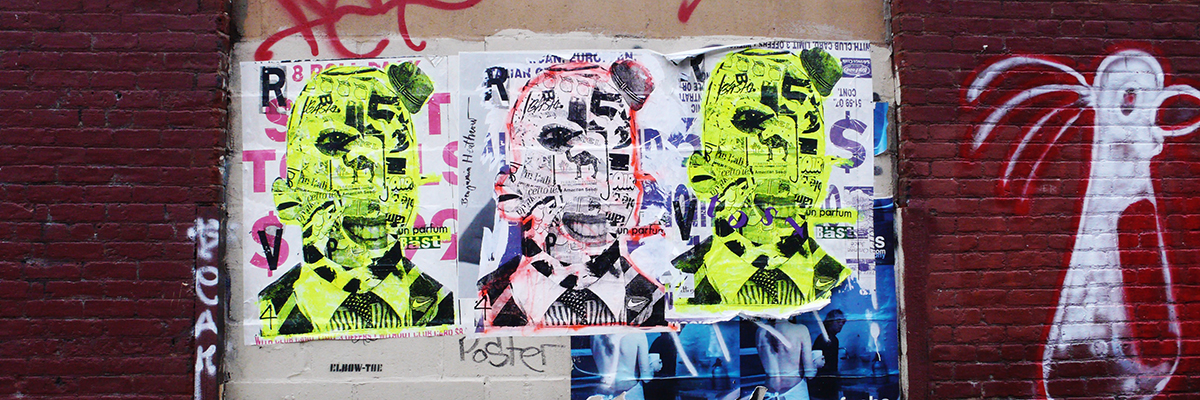The image depicts a heavily graffitied wall composed of dark red-painted brick. Prominently featured are three visually striking posters, each showcasing a composite image of a bald man wearing a hat and a black suit with a white collared shirt and tie. The posters are constructed from various magazine cutouts, including mismatched eyes, mouths, and a small camel representing the nose. Two of the posters are accented with yellow-green hues, flanking a central poster highlighted with a white background and a red border. Above each head, text partially spells out "R... T." The chaotic aesthetic is complemented by extensive graffiti, including a large, abstract white bird-like figure on the wall's right side, painted in a manner that allows the red brick to show through in sections. The overall scene conveys a gritty, urban street vibe with layers of text and paint interwoven with the posters and graffiti.